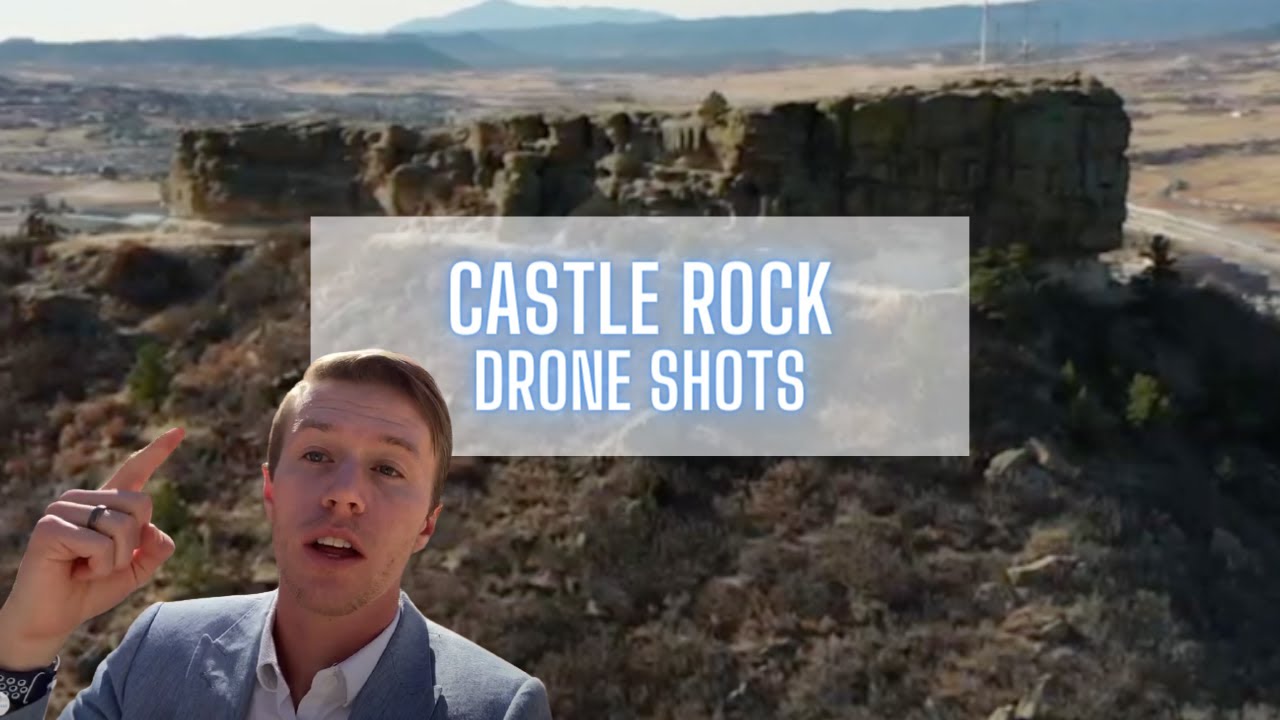In the detailed aerial photograph of a large mountainous plateau, captured most likely by a drone, the rugged terrain unfolds with striking clarity. Dominating the center, the plateau is characterized by its rocky structures and varying vegetation, displaying a harmonious blend of browns, grays, and greens. A slope encircles this majestic rise, adorned with patches of grass and clusters of local flora. In the far background, additional mountains and a tall, white telephone pole are faintly visible, further enriching the dramatic landscape.

In the very bottom left corner of the image, a man is superimposed, likely through green screen technology. He is visible from the shoulders upwards, attired in a gray business coat over a white button-up shirt with the collar slightly undone. Wearing a black ring on his ring finger and a black wristband on his watch, he points upwards towards the plateau, seemingly discussing the scene. Overlaid on the image is a semi-transparent white rectangle with white text bordered in blue, bearing the caption "Castle Rock Drone Shots." The photograph, taken in broad daylight, bathes the entire scenery in natural sunlight, enhancing the vivid details of both the landscape and its digital augmentations.